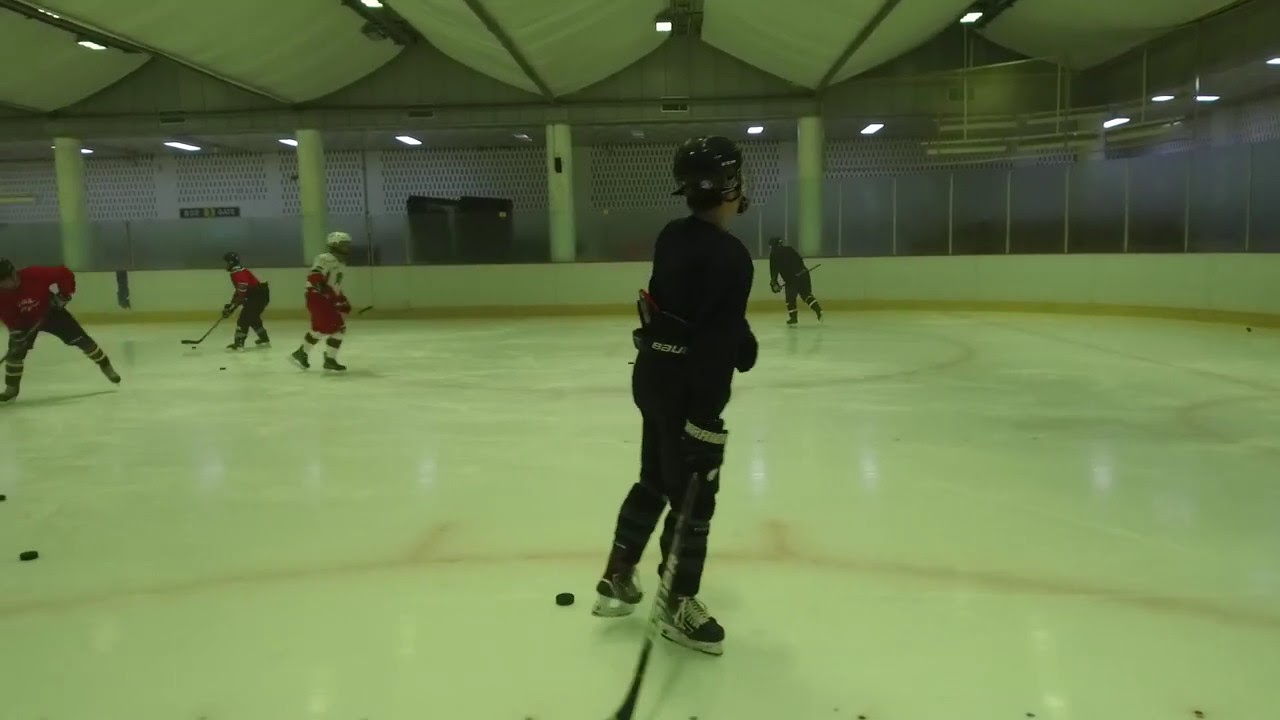The image captures an ice hockey practice session inside a stadium from the perspective of someone on the rink. The scene features five players dressed in full gear – three in red jerseys and two in black. The players are scattered with several pucks on the ice, indicating a practice environment rather than an ongoing game. 

In the center, a player in red, with his back towards the viewer, appears to be skating to the right. To his left, near a puck, stands another player in black gear, also looking away from the puck. On the left side of the image are two more players in red jerseys with black helmets, slightly crouched and seemingly poised to take action. Nearby, an additional player in black is visible near the rink’s wall, skating towards the left. One player in white, also holding a stick close, is heading towards the right of the rink.

The rink itself is surrounded by walls with glass paneling, and the ceiling features curved patterns with lighting fixtures around the edges. Red markings, including circles and lines, are visible on the ice, contributing to the structured environment of the practice session. The empty stands in the background further reinforce the atmosphere of a training exercise rather than a competitive match.